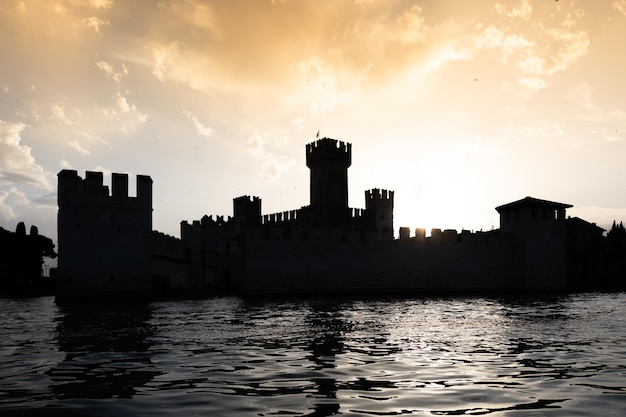The photograph showcases a majestic castle set against a dramatic and colorful sky. The sun is either rising or setting behind the structure, casting it and the surrounding complex in deep shadow and making the entire scene appear almost black. The sky is an artistic blend of bright pink, yellow, and shades of white and yellowish-brown clouds. The castle, although largely silhouetted, reveals intricate battlements with jagged, tooth-like edges atop its walls and at least one round turret. Adjacent to the castle is a smaller house, and some trees are visible nearby. The foreground features dark, nearly black water with silver or white waves, reflecting the castle’s shadowy outline. In the distant right side of the image, a faint silhouette of a mountain can be seen, adding to the picturesque and moody atmosphere.